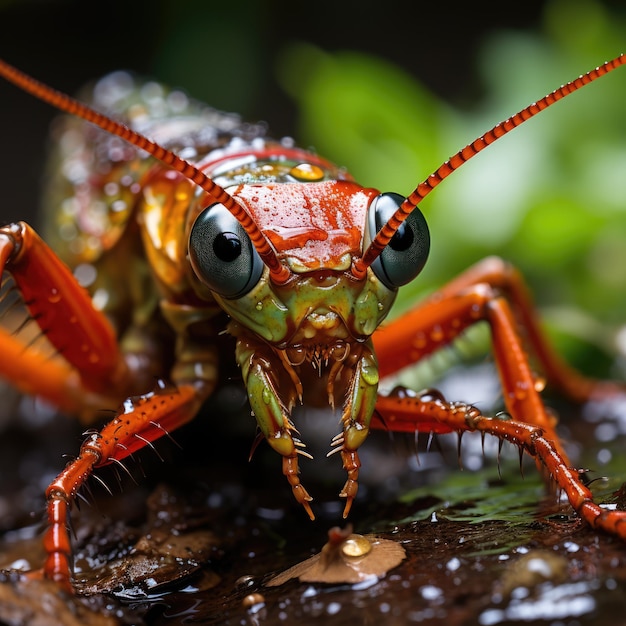This close-up photograph features a vibrant grasshopper-like insect, predominantly red and green, showcasing remarkable detail on its body and surroundings. The insect's head and front legs are distinctly reddish-orange, with large, bulging eyes that exhibit a black and gray hue with prominent black pupils. Two long, reddish-orange antennae extend towards the corners of the image, adding to its striking appearance. Notably, the insect's small brown pincher claws protrude from its mouth region, contributing to its aggressive demeanor.

Its reddish-orange legs are emphasized, appearing slightly hairy, while the remaining legs fade out of focus, merging with the blurred background. The background itself is a mix of green and brown, with hints of moist, faded leaves suggesting a damp forest floor, possibly after rain. The insect's body, reminiscent of a lobster, and its slender form are partially visible, tapering into a hazy abdomen. The insect stands on what appears to be a wet, brown and green leaf or rock, adorned with water droplets, suggesting an environment rich in moisture. Overall, the intricate textures and vibrant colors create a vivid, engaging portrayal of the insect in its natural habitat.